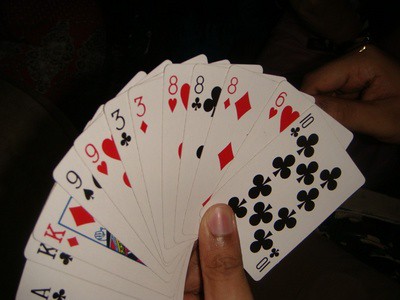In this image, we are looking at a detailed view of a hand of playing cards fanned out against a predominantly dark background. The foreground reveals a thumb and finger holding the cards, which appear slightly worn from use, with visible handling on the corners and edges. The fan of cards consists of an ace of clubs, two kings (one of clubs and one of diamonds), two nines (one of spades and one of hearts), two threes (one of clubs and one of diamonds), three eights (one each of hearts, clubs, and diamonds), a six of hearts, and a ten of clubs. The cards are clearly grouped, suggesting the player might be organizing them for a game like rummy. In the upper right corner of the frame, there is a faint image of another player's hand, implying an ongoing game. The background remains mostly black, emphasizing the fanned out hand of cards in the foreground.